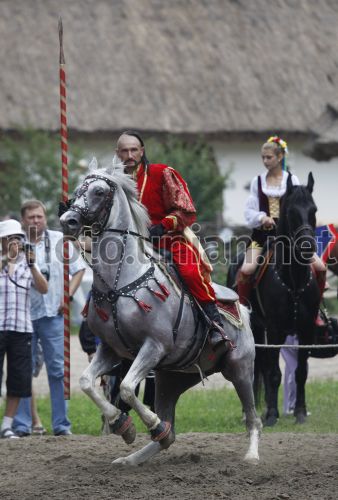In this image, a striking scene unfolds at what appears to be a Medieval Times or Renaissance-themed event. A man, dressed in a vibrant red costume resembling a jester's attire, rides a white-gray horse adorned with red tassels and chains on its harness. The man sports a distinctive hairstyle, shaved on one side and long on the other, and holds a bright red and yellow striped spear. Following him is a young woman on a black horse, donning a period-appropriate Renaissance costume which includes a corset (or boussier), a white ruffled shirt, and a flowing skirt. She also wears a crown of flowers in her hair, adding to the authenticity of her outfit. Behind them, people dressed in contemporary attire can be seen taking photographs, while trees decorate the distant background. The image is also marked with text, though partially illegible, suggesting a watermark of "o-h-o-t-o dot u-n-i-a-n dot n-e-t." The entire scene evokes an old-fashioned spectacle, rich in historical attire and atmosphere.